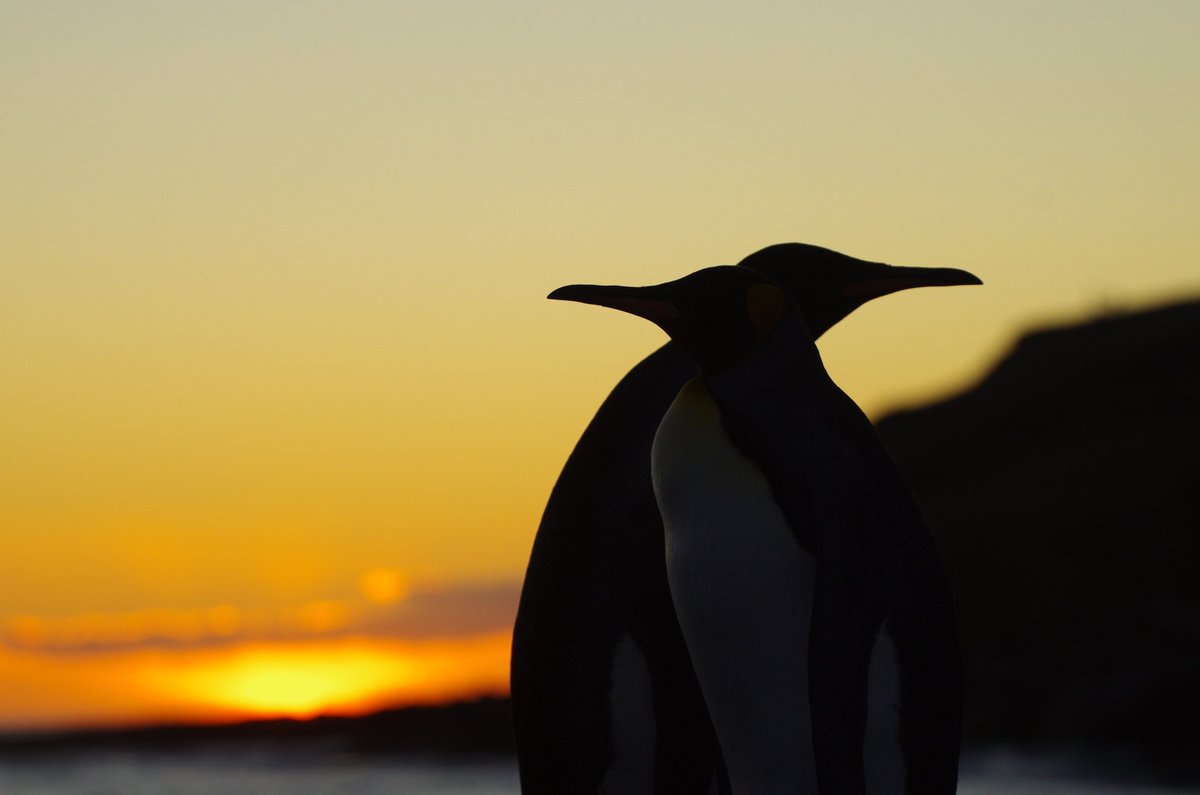In this professionally staged, full-color photograph, the outdoors scene captures a stunning sunset that bathes the sky in a gradient of yellow and orange hues. The horizontally rectangular image places the setting sun in the lower left-hand corner, just a bright glow not fully visible yet. Above the sun, thin orange clouds merge into darker ones as the sky stretches upward.

Dominating the composition just to the right of the center are two adult penguins silhouetted against the colorful sky. They stand back-to-back, their heads and bodies in shadow, their beaks pointing in opposite directions. The penguin on the right is slightly closer to the camera, revealing a faint hint of its white and orange belly where the shadows soften. Despite the lack of detailed features, the distinct shapes and neck positions clearly identify them as penguins.

The background remains blurred, focusing all attention on the penguins' intimate pose. To the right of the birds, a dark landmass or hill outcropping fades into the shadowy part of the scene, enhancing the serene and slightly mysterious atmosphere of this meticulously captured moment.